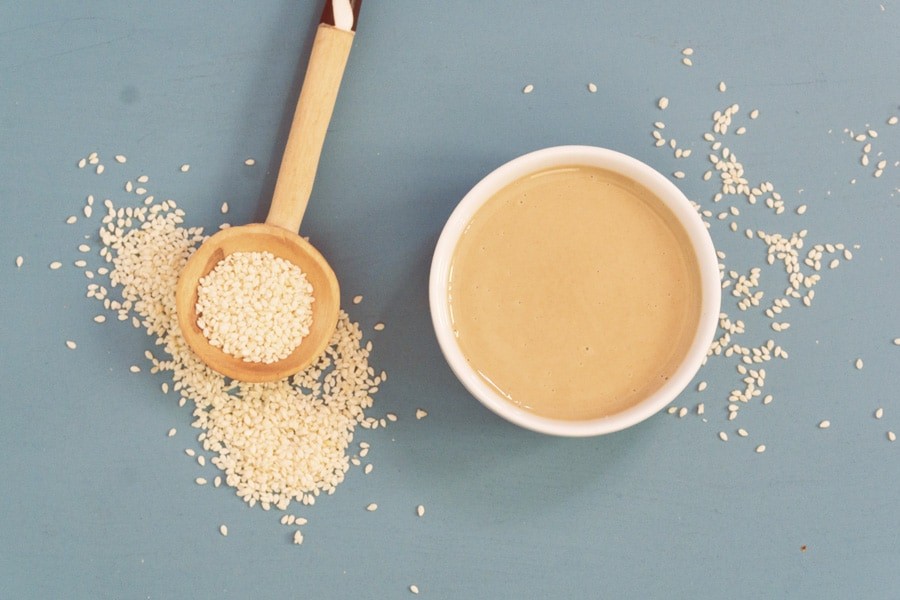The image depicts a shallow white bowl filled with a light beige, creamy liquid, likely tahini, situated on a light teal surface. Scattered across this surface and partly immersed in the liquid are numerous sesame seeds. A broad wooden spoon, filled with sesame seeds, lies atop the teal surface and partially submerged in the bowl's liquid. The spoon’s wide base is complemented by the thin, creamy texture of the liquid, reminiscent of coffee with creamer. The scene includes some stains on the surface, adding a touch of rustic authenticity.